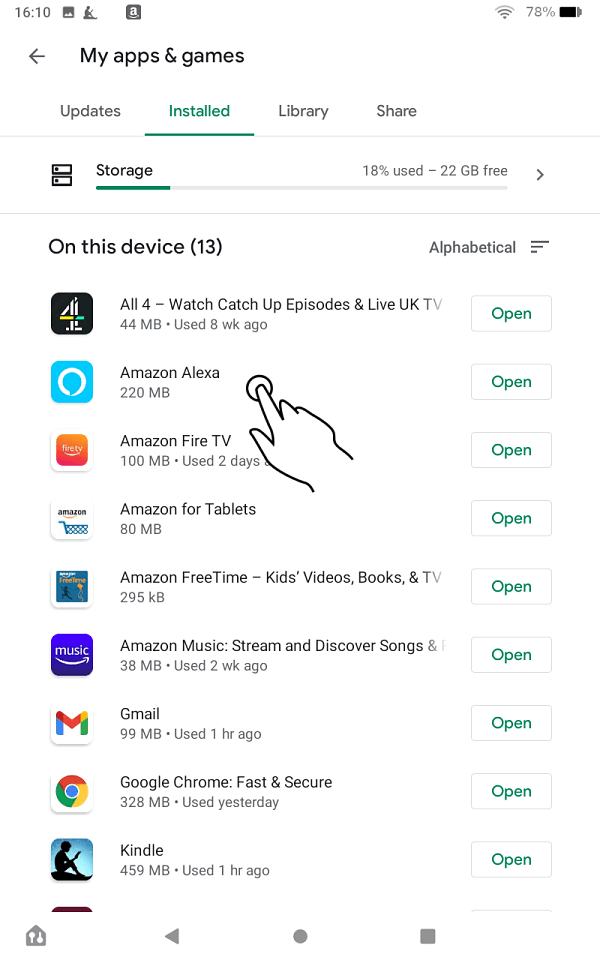The screenshot displays the "Installed" menu of the Google Play Store app on a tablet. At the top of the screen is the Android status bar, which shows the time as 16:10, followed by a screenshot icon, an icon of a person sitting, a blank icon, and an Amazon app icon, all displayed in dark grey. On the far right, there is a Wi-Fi icon and a battery indicator showing 78% charge.

At the bottom, the Android navigation bar features the back, home, and recent apps icons, represented by a triangle, circle, and square, respectively.

The main part of the screen is titled "My Apps & Games" in black text, with a back arrow to its left. Below the title, there are four tabs: Updates, Installed, Library, and Share. The "Installed" tab is highlighted in green, indicating it is currently selected.

Directly underneath the tabs is a horizontal divider, followed by a storage usage summary. It shows a green bar indicating that 18% of storage is used, with 22GB free.

Further down, the section titled "On This Device" reveals there are 13 installed apps, sorted alphabetically, with a sort button available. Listed apps include:

1. Watch Catch-Up episodes and Live UK TV
2. Amazon Alexa
3. Amazon Fire TV
4. Amazon for Tablets
5. Amazon FreeTime (Kids Videos, Books, and TV)
6. Amazon Music (Stream and Discover Songs)
7. Gmail
8. Google Chrome (Fast and Secure)
9. Kindle

Each app entry displays the app icon on the left, the app name in the center, the app size below the name, and an "Open" button on the far right. Central to the screen, there is a black clip art image of a hand tapping the screen, illustrating interaction.